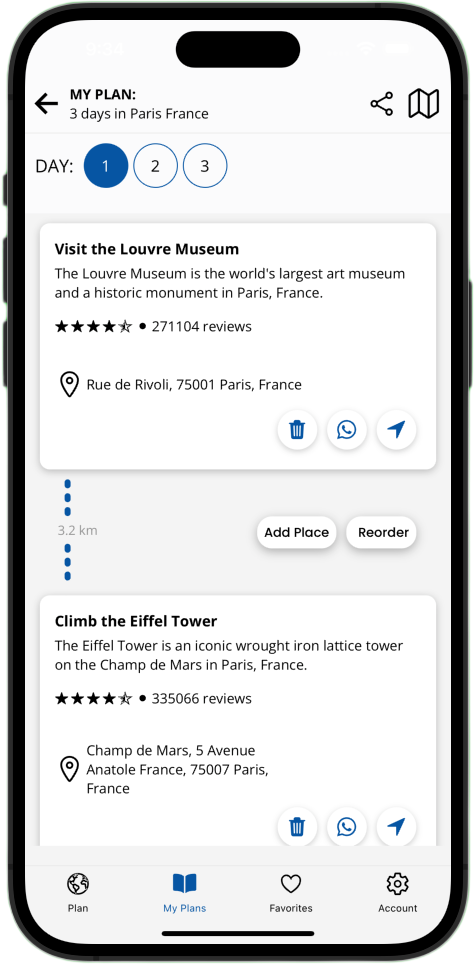The image displays a cell phone with a black outline, set against a pale grey background. The cell phone screen is open, displaying a travel planning application. At the top of the screen is a back arrow icon, followed by the title "MY PLAN" in capital letters and small font. Beneath that, in larger font, it reads "Three days in Paris, France". Moving to the right on the same line are a map symbol and an interconnected circles icon.

Directly underneath, the app labels the current selection as "Day:", followed by three numbered circles (1, 2, and 3). The first circle (1) is filled in blue, indicating the current selection. Below this, in a white rectangular block, there is an itinerary item: "Visit the Louvre Museum", accompanied by some brief information about the Louvre and its address.

Further down, the screen displays a series of three dots, followed by the distance in kilometers, then three more dots leading to the next itinerary item: "Climb the Eiffel Tower".

At the bottom of the screen, there are three navigational icons: a globe that reads "Plan My Places" with a book symbol above it, "Favourites" with a heart symbol above it, and "Account" with a settings gear icon.